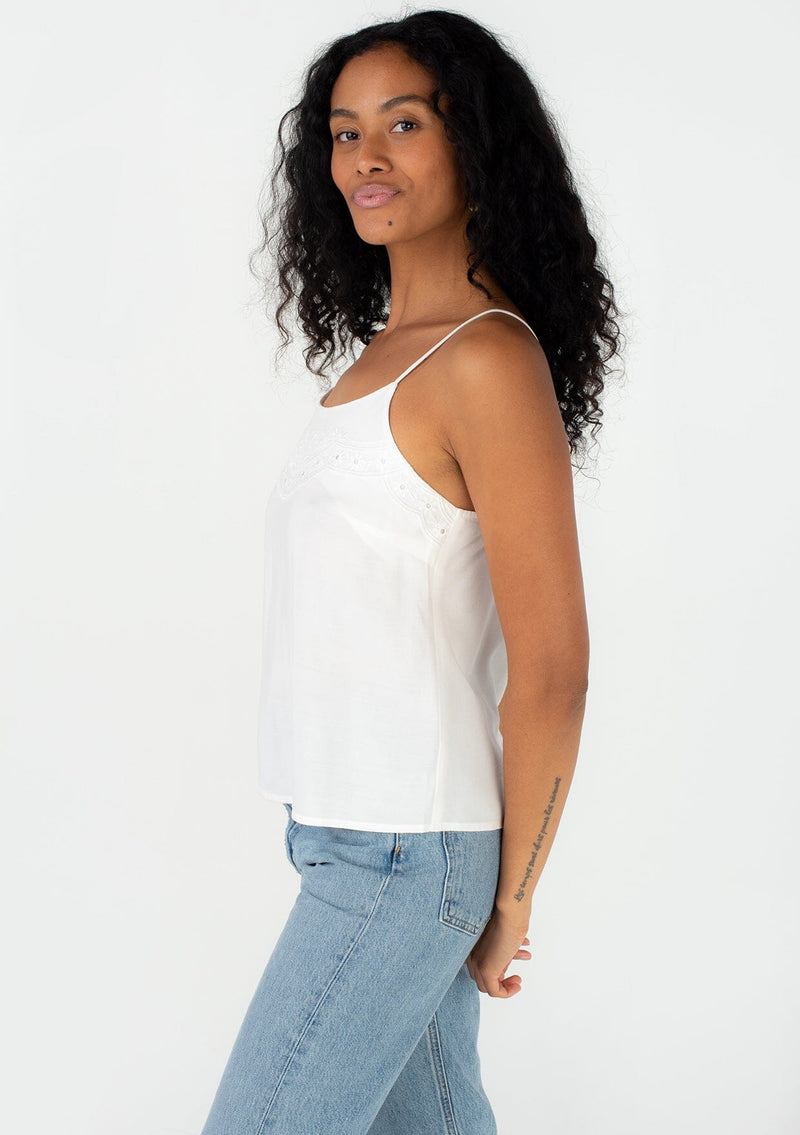The photograph captures a young model standing confidently against a plain white wall, emphasizing her striking presence. The portrait-oriented shot features a brown-skinned woman, possibly African-American, with flawless complexion and long, wavy black hair cascading down to the middle of her back. She strikes a strong pose with her left shoulder angled towards the viewer and her hands behind her back, her face turned towards the camera with a cheeky expression, slightly raised eyebrows, and a playful pout accentuated by bright pink lipstick. Her attire is casual yet stylish, consisting of a plain white vest-style tank top and light-colored jeans, suggesting she might be modeling for a clothing brand or fashion magazine. Additionally, she has a distinctive small black tattoo with words on her left forearm and a mole on her lower left chin, adding to her unique and captivating appearance.